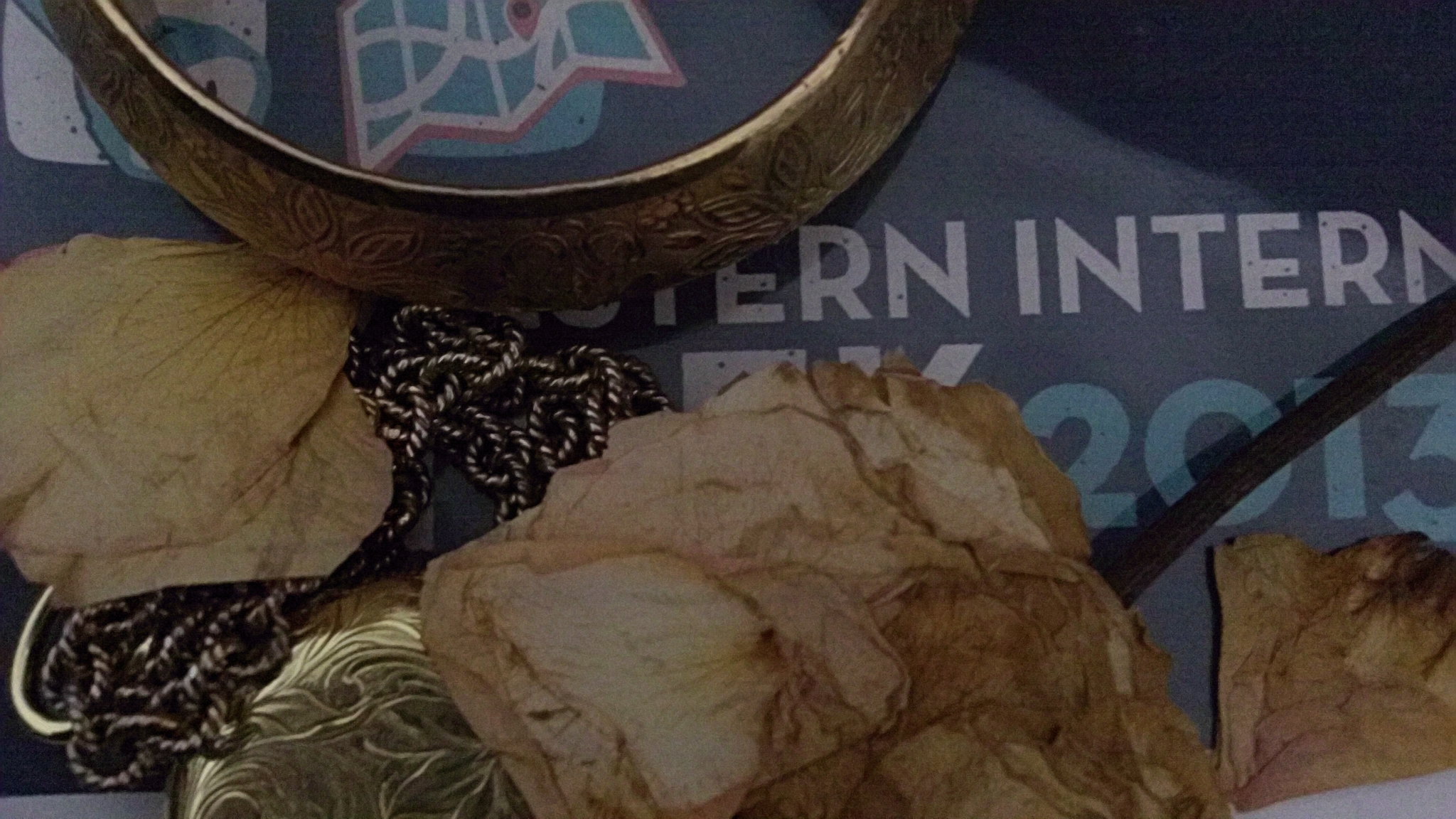The photograph features an assortment of items displayed on a blue background with partially obscured text that possibly reads "Western Intern 2013." Prominently, there is a golden, oval-shaped metallic object, which might be a picture frame or a large ring. Adjacent to it is a silver piece that could be a bracelet or a long, thin chain resembling a rope. Also in the scene, there are brown wrapping materials, either crumpled rags or aged paper, tied together with twine. These items are placed on a glass-topped table, contributing to the unconventional and eclectic composition of the image.